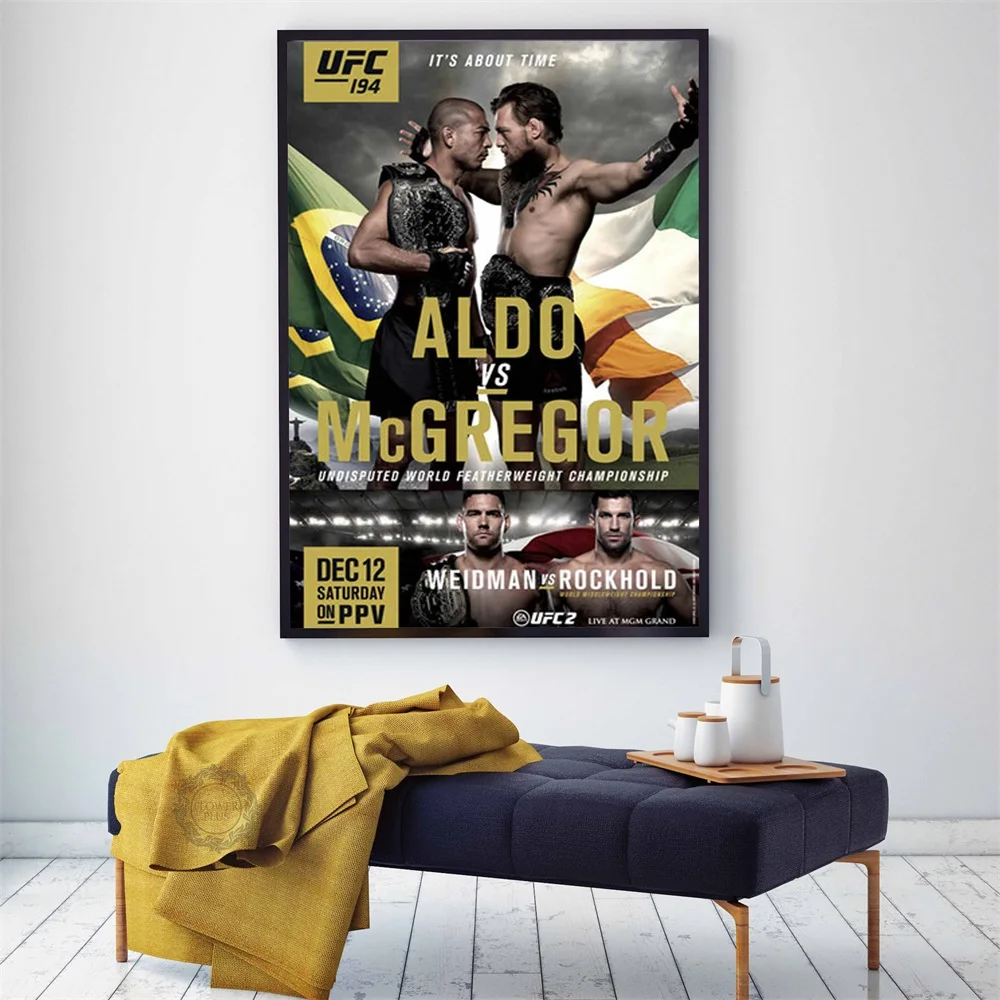This image depicts a modern and minimalistic room with white walls and wide plank, white hardwood floors. A blue upholstered chair with wooden legs sits prominently in the foreground. Draped over the left side of the chair are yellow blankets or towels, while on the right side rests a light brown tray holding three white containers. Behind the chair, a framed UFC poster stands out against the white wall. The poster showcases a cloudy gray sky background with the bold text, "It's About Time UFC 194", featuring two men facing off, one holding a belt and the other wearing one. The contenders, Aldo and McGregor, are competing for the undisputed World Featherweight Championship, scheduled for December 12, Saturday on PPV. Adding a pop of color to the room, the poster integrates a color scheme of black, white, gray, yellow, blue, green, red, gold, tan, and brown.